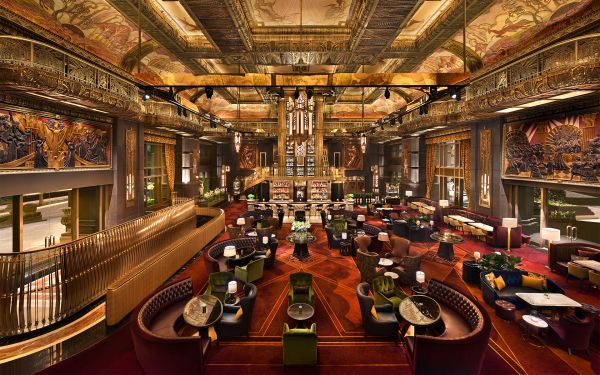This photograph captures an opulent and expansive dining hall, reminiscent of a high-end lounge with elements suggesting a mid-20th-century design. The room is characterized by its towering ceilings adorned with intricate, cathedral-like murals and ornate gold decorations. The floor is covered with a reddish-brown carpet featuring geometric patterns and white engravings, enhancing the luxurious feel of the space. Plush seating arrangements, including round and varied tables paired with brown and green velour chairs, add to the upscale ambiance. On either side of the room are large windows that flood the space with light. The focal point appears to be a grand bar area at the far end, adorned with a golden structure reminiscent of a cathedral facade, flanked by a combination of studded leather benches and cushioned chairs, reinforcing the sense of a ritzy, sophisticated establishment.